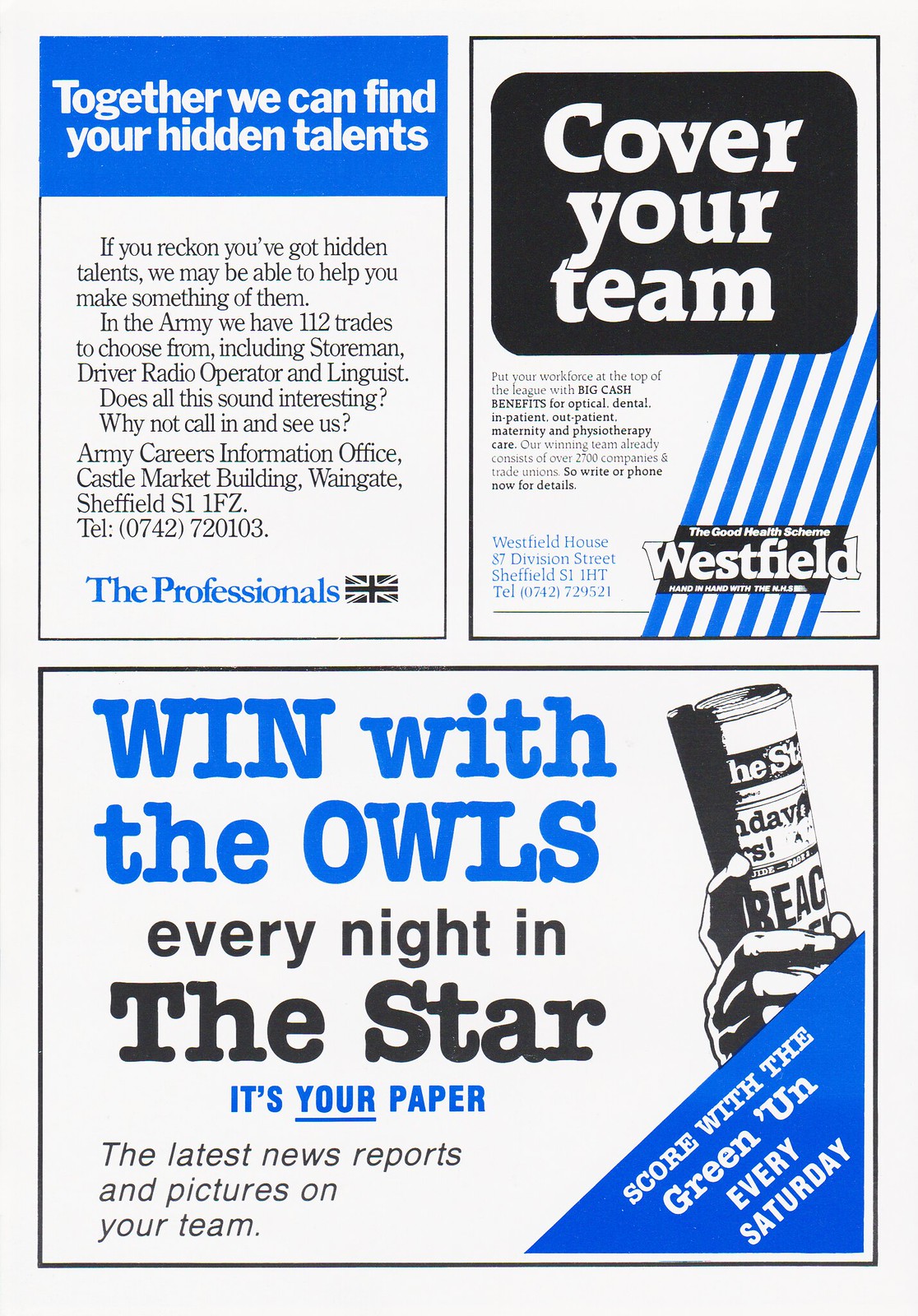The image features a detailed advertisement page resembling a newsletter, with a white background and is divided into three primary sections. The top-left quarter of the page displays a blue bar with white text that reads, "Together we can find your hidden talents." Below this, additional text invites potential recruits to explore their hidden talents with the Army, offering up to 112 trades such as storeman, driver, radio operator, and linguist. The contact details for the Army Careers Information Office in Sheffield are prominently provided.

Adjacent to this, the top-right quarter features an advertisement with the headline, "Cover your team" set against a background with black and blue graphic elements. The specific messaging within this section is indistinguishable, but it is suggested to bear relevance to team coverage, possibly sponsored by Westfield.

Spanning the bottom half of the page, another rectangular advertisement in bold blue text declares "Win with the Owls." It continues, mentioning "every night in The Star, it's your paper," indicating a newspaper promotion that includes the latest news reports and pictures of the team. At the bottom-right corner, a blue triangle highlights the phrase "Score with the Green ‘Un every Saturday," accompanied by an illustration of a hand holding a newspaper.